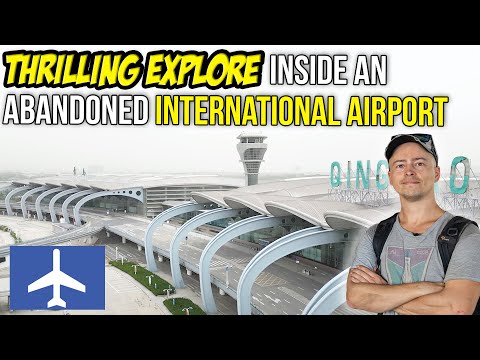This image is a YouTube thumbnail for an exploration video titled "Thrilling Explore Inside an Abandoned International Airport." The text, prominently featured, includes "Thrilling Explore" in yellow with black shading, "Inside an Abandoned" in white with a black border, and "International Airport" in yellow with a black border. In the image, a Caucasian man wearing a gray t-shirt with backpack straps, a camouflage hat, and a smile stands with his arms crossed in front of his chest. Behind him is the expansive, modern, and seemingly abandoned Qingdao International Airport terminal. The terminal features large, curving roadways bordered by steel archways and a sophisticated, white-colored ceiling. Visible through the glass windows of the terminal is the aircraft control tower, centrally located in the background. The lower left corner of the thumbnail includes a small blue square tile with a white airplane silhouette. Above the man, partially visible green letters "Q, I, N, C," and ending with "O" appear superimposed, adding a mysterious element to the visual.